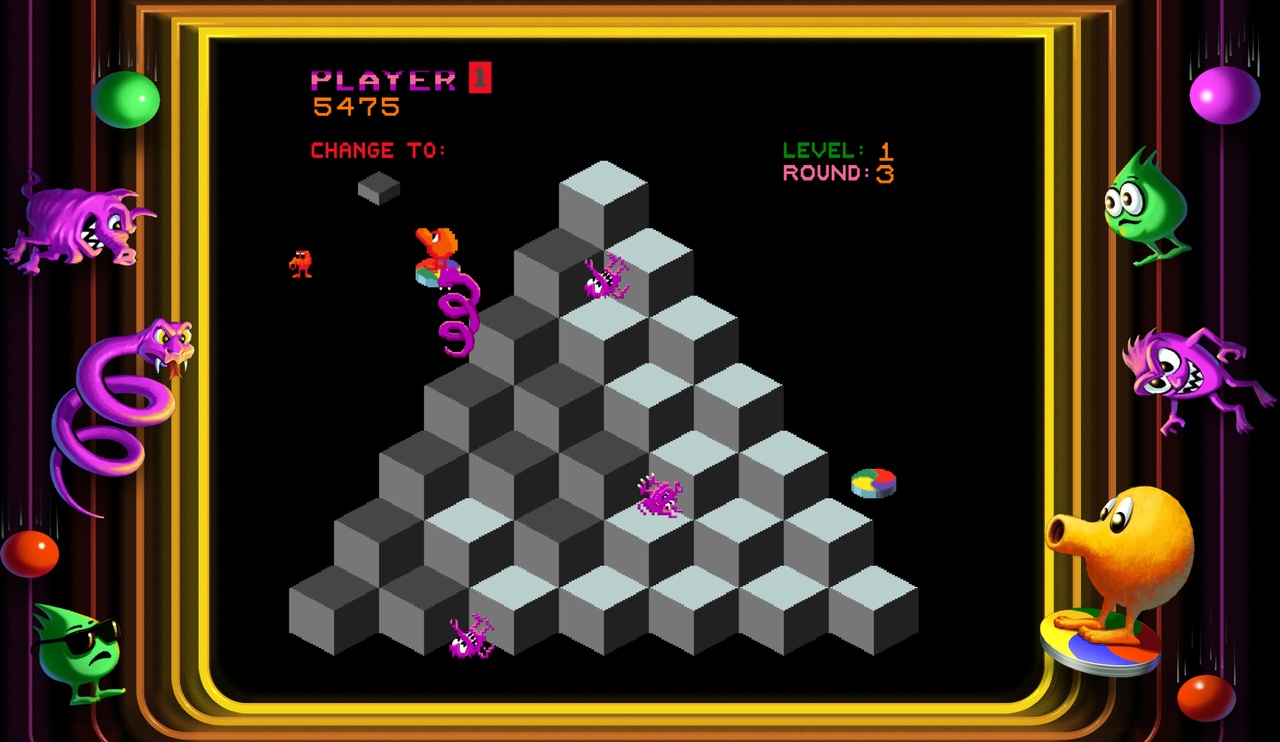The image depicts a vintage video game screen, likely from around 20 years ago or slightly newer. Dominating the center is a pyramid-like structure composed of gray and white blocks. Surrounding this central pyramid are various cartoon-like characters scattered around the border. 

Details include:
- At the top of the screen are the indicators "Player 1" with a score of 5475, followed by "Level 1 Round 3."
- Along the border, starting from the bottom left, is a small green character wearing black shades.
- Above this character is an orange ball, followed by a purple swirly snake, a pink monster resembling an angry pig, and another green ball.
- On the right side, the sequence features a small green character, a purple monster, and an orange character with a tube-like mouth standing on a multicolored disc.
- The pyramid itself is occupied by additional small critters, including a red creature with an elephantine snout and feet, and several purple pig-like monsters with sharp teeth. The purple snake is also positioned somewhere on the pyramid.

Overall, the screen showcases the retro game’s vibrant and quirky artistic design, emphasizing its playful combination of colorful, distinct characters and geometrical gameplay elements.